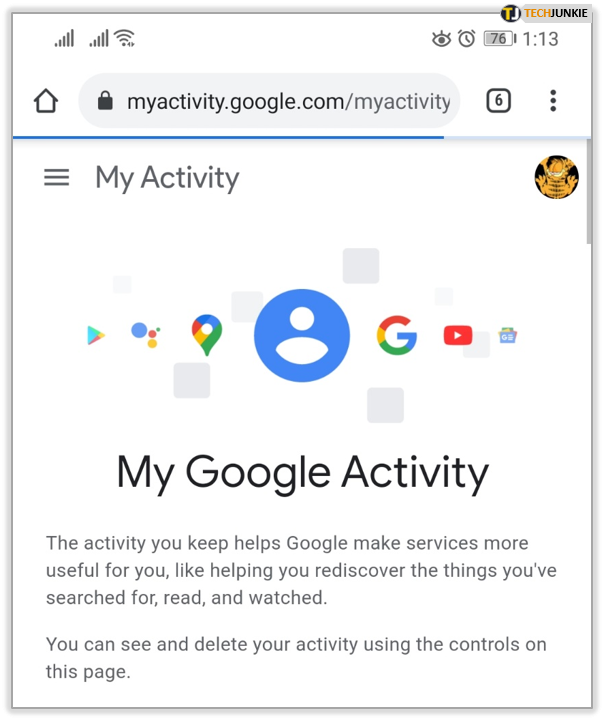This vertical mobile screenshot captures a detailed view of a phone's screen. In the top left corner, the image shows two full service bars and an active Wi-Fi icon; meanwhile, the top right corner displays the eye icon for an alarm, a battery level at 76%, the time "1:13", and a watermark from "Tech Junkie" featuring a circular logo with yellow "T" and white "J". The primary content of the screenshot illustrates a Google search bar positioned at myactivity.google.com/myactivity.

Below the search bar, the text "My Activity" appears on the left, adjacent to three horizontal lines (menu icon). On the right, there is an icon resembling Garfield with a black background, his arms and legs spread out and an expression conveying smugness.

In the central portion of the image, a blue circle with a user icon is visible, followed by several application icons including Google Chrome, Maps, Google Play, YouTube, and Gmail. The impact of "My Activity" is described in black text: "The activity you keep helps Google make services more useful for you, like helping you rediscover the things you've searched for, read, and watched. You can see and delete your activity using the controls on this page." A thin gray border encapsulates the entire image.